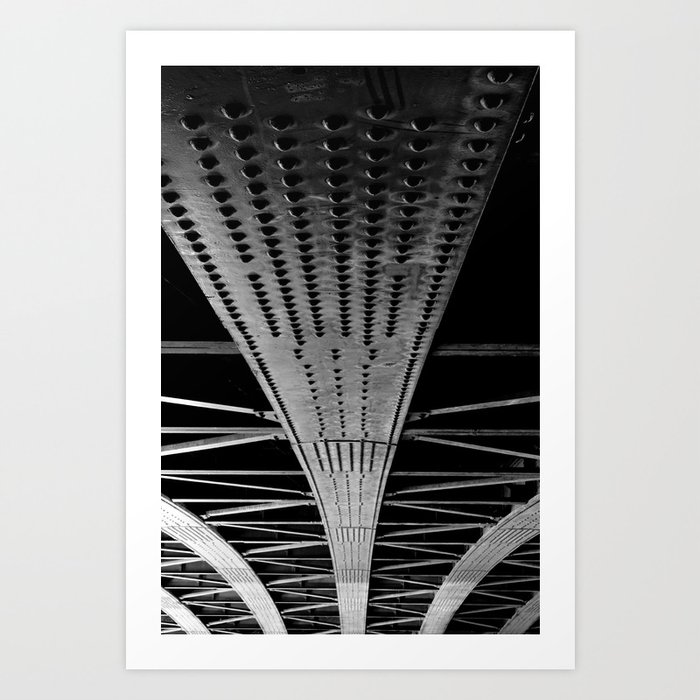This black and white portrait-oriented photograph appears to depict the underside of an industrial bridge, with a focus on its architectural elements. The background of the photo is predominantly black, interspersed with horizontal gray stripes, creating the impression of an expansive, inverted triangle expanding outward from the center. At the core, a prominent central beam is flanked by pairs of smaller steel beams, all held together by hundreds of visible metal bolts. The beams extend diagonally to the left and right, accentuating the structural intricacies. This photograph, possibly mounted on a gray wall, includes a white border, suggesting it might have been captured as an artistic or poster-style image.